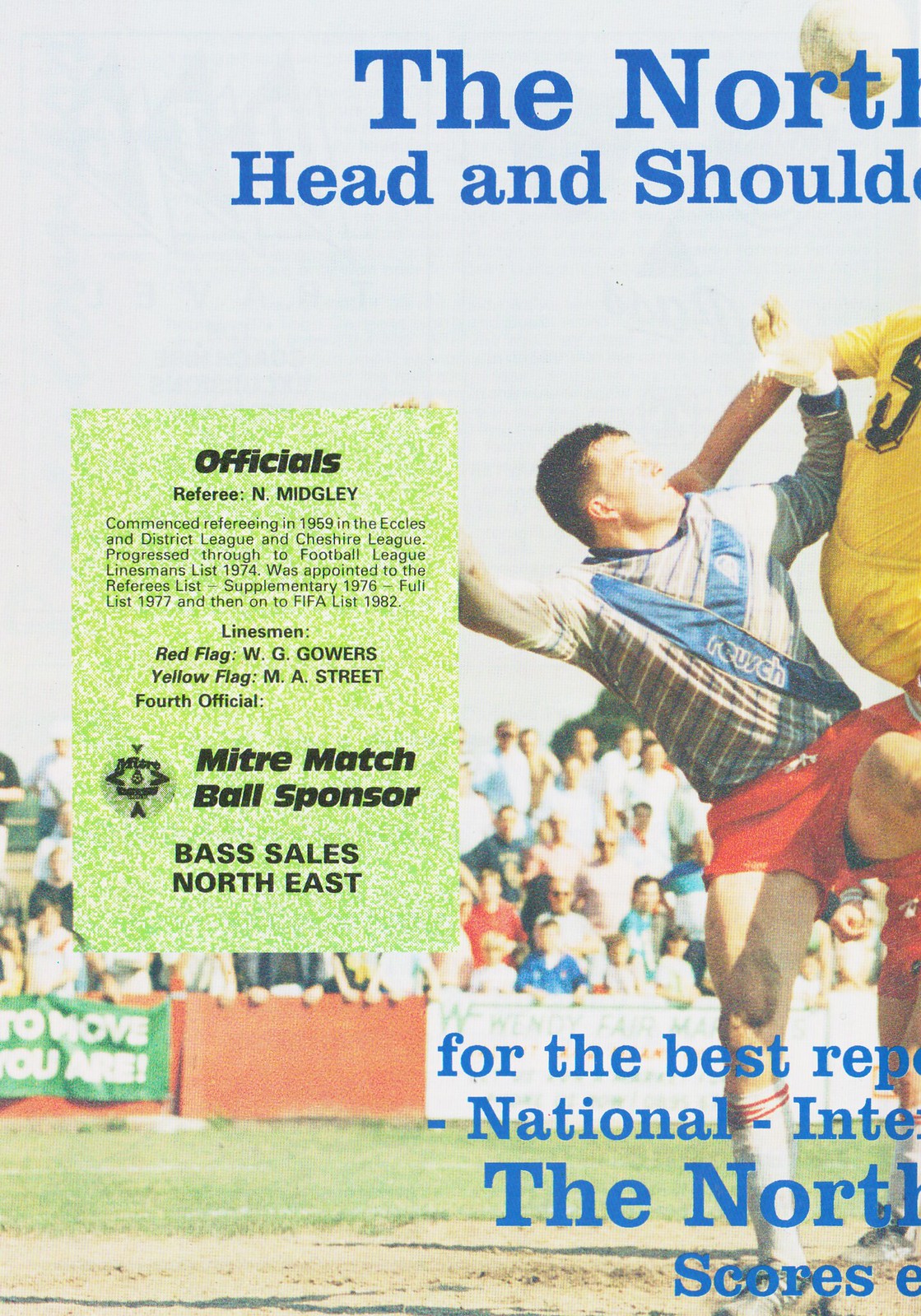The image depicts the front cover or a page from a game day program or magazine, primarily featuring a sporting event, likely soccer or possibly rugby. Dominating the center is a photograph of two players competing for possession of the ball, set against an outdoor backdrop indicative of a stadium setting, with visible green grass and patches of dry dirt. One player is dressed in a gray and blue jersey paired with red shorts and white socks, while the other player sports a yellow jersey with matching yellow shorts.

At the top of the page, partially cropped blue text reads "The North Head and Shoulder Officials Referee N. Medley," detailing his career progression from local leagues to the Football League since 1959 and his listing as a linesman in 1974. The bottom also features blue text, similarly cropped on the right side.

On the left side of the page, there is a green rectangular box with black text listing the officials, including the referee, linesmen, and the fourth official. Also mentioned is a sponsorship by Mitre Match Ball Sponsor Bass Sales Northeast. The image utilizes a vivid color palette, featuring shades of gray, blue, green, white, black, yellow, red, and orange, contributing to its dynamic and engaging composition.